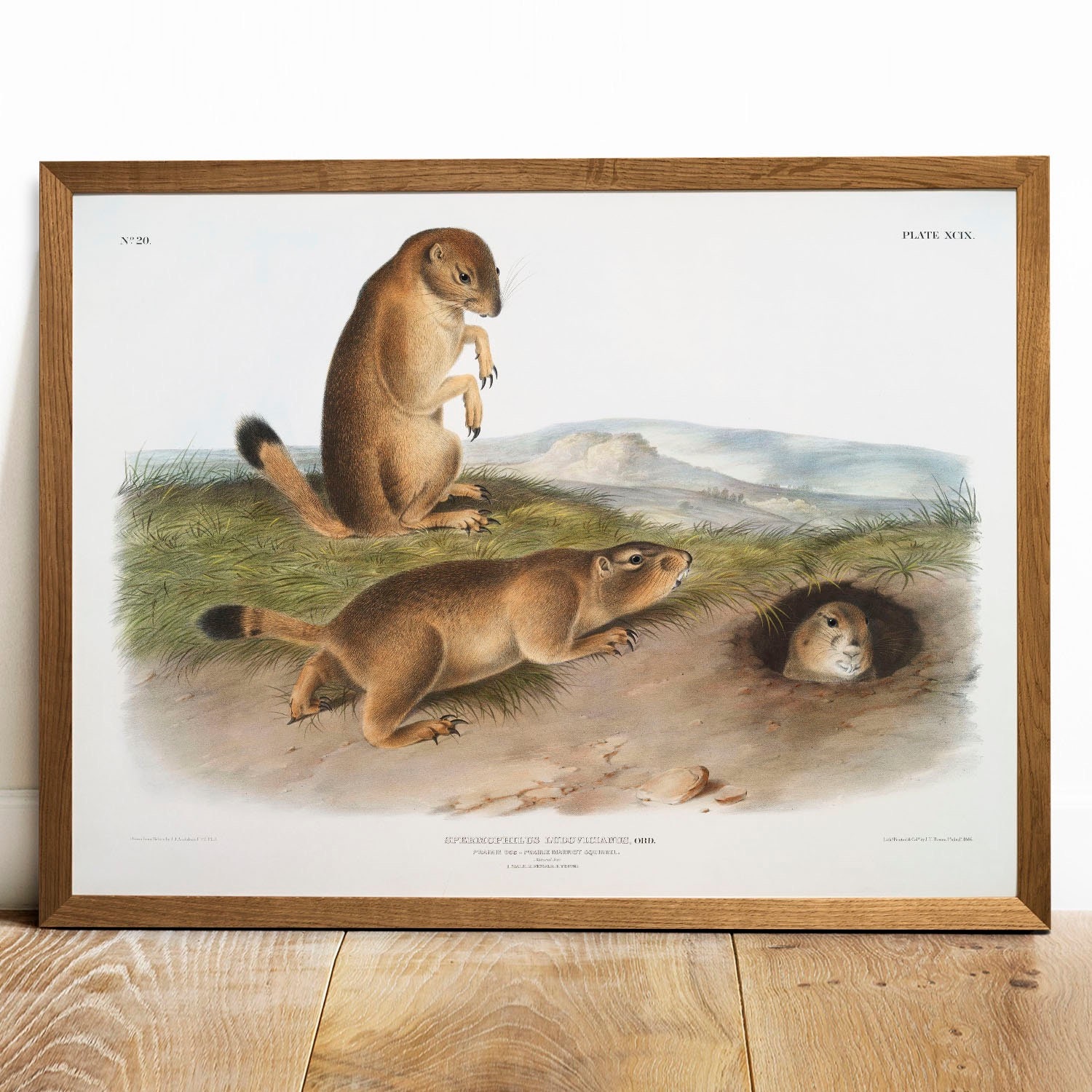The image depicts a framed illustration of ground squirrels, positioned on a wooden floor with three wide planks, leaning against a white wall in an indoor setting with probable artificial lighting. The frame is a similar shade of light brown wood and is not very thick. The picture itself, oriented in landscape, shows a detailed and realistic representation of a natural scene. 

In the illustration, there are three ground squirrels: one larger squirrel is standing on its hind legs, displaying its long claws, while another is on all fours approaching a hole. From this hole, the third squirrel can be seen peeking its head out. The background features dirt, grass, and hills, enhancing the wilderness setting. 

The artwork contains small, illegible text in the upper right corner, a number in the upper left corner, and additional writing at the bottom center, which also cannot be read. The entire image is captured in a full-color photograph, casting a slight shadow on the left side of the wall behind it.